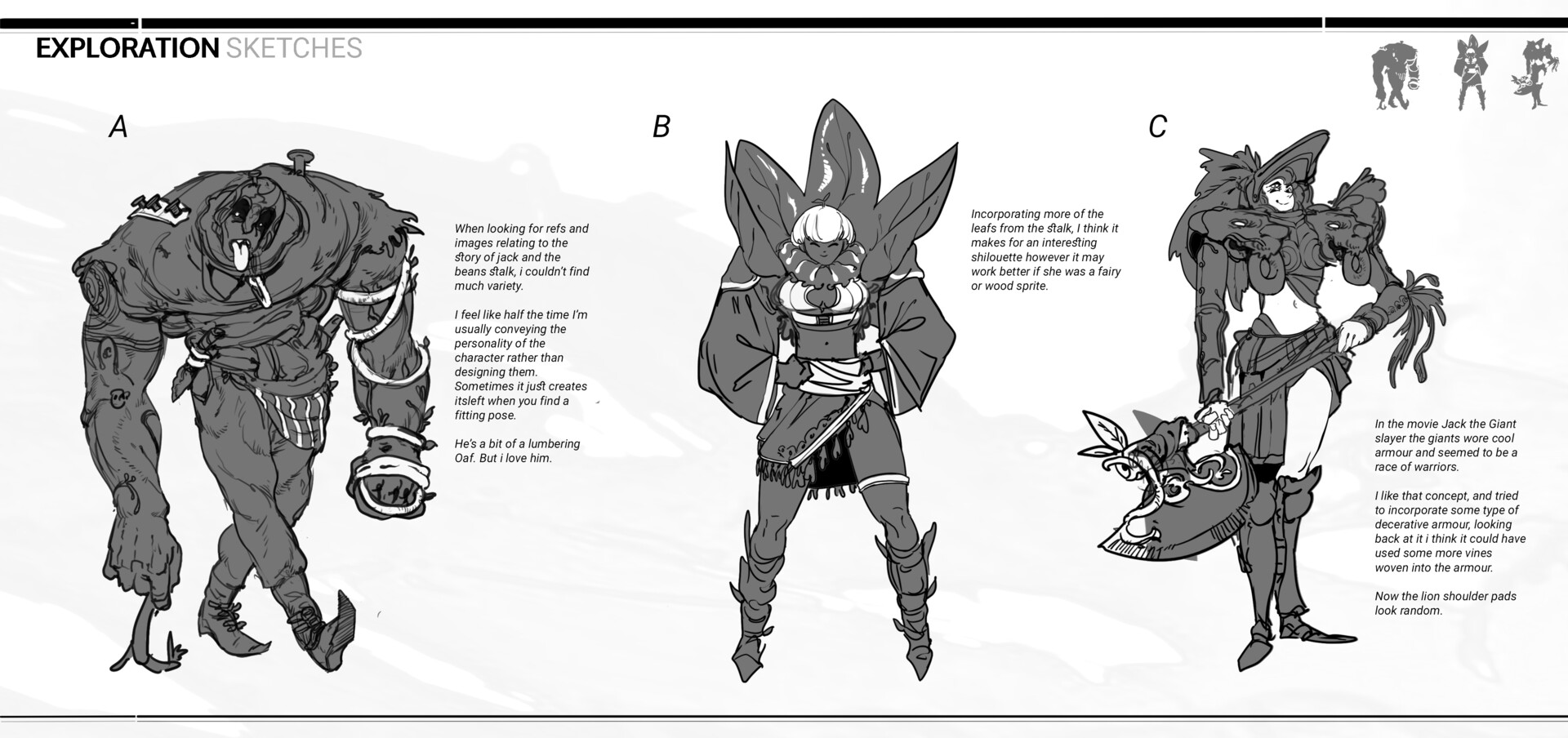This is a black and white pencil-colored page labeled "Exploration Sketches," featuring three character designs inspired by "Jack and the Beanstalk." Character A, situated on the far left, is a large, grotesque male figure with bedraggled clothing and pointed shoes. He is described as a lumbering oaf with deep black eye sockets and a tongue lolling out. His bulky frame contrasts with his skinny legs, and he has a hook-like appendage on his right hand while his left hand is bandaged. Character B, placed in the middle, is a unique female figure with leaves sprouting from her neck and leafy petals extending from her back, resembling wings. She wears a short skirt and pointy shoes, with beads adorning her neck, giving her a mystical, wood-spirit appearance. Character C, on the right, appears to be Jack himself, dressed in a mix of decorative armor and practical clothing. He sports lion-shaped shoulder pads, a pointed hat, and knee-high boots. Holding a large battle axe in both hands, his bare belly adds an unusual touch to his formidable look. This collection of sketches presents a vivid exploration of characters that are both fantastical and detailed, staying true to the whimsical yet intimidating essence of the story.